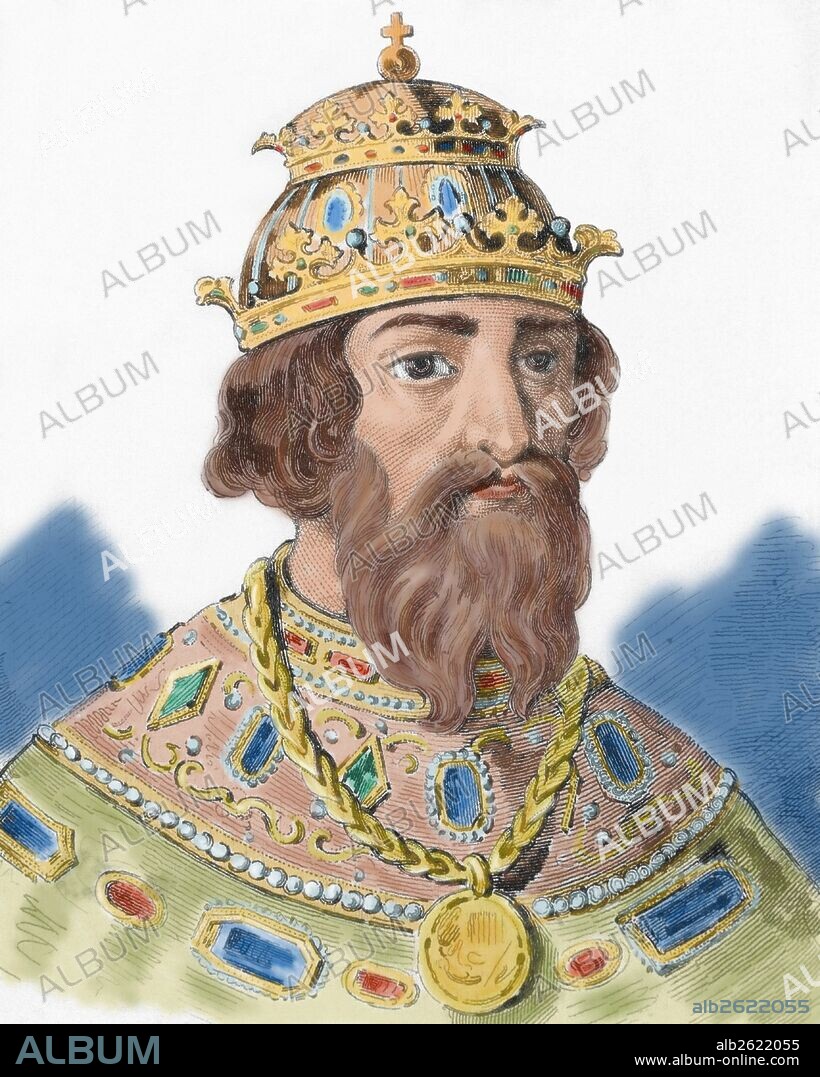The image is a detailed watercolor-style drawing of a regal figure, possibly a king or a religious leader from late medieval Europe, potentially from the Slavic regions. The central figure is a bearded man in his 40s, with long, wavy brown hair covering his ears and a moderately long, blonde beard reaching his collarbone. He is adorned with an ornate, upside-down soup tureen-like gold crown encrusted with jewels and topped with a gold ball and cross.

His head tilts slightly to one side, projecting a noble demeanor. He wears a cream-brown and light green frock with a round neck and an elaborate collar that elegantly curves from his left shoulder to his right. This frock is embellished with a row of large, colorful jewels extending diagonally across his chest. Draped around his neck is a heavy gold chain supporting a substantial gold medallion.

Throughout the illustration, the word "ALBUM" appears as a watermark, and across the bottom, a black bar displays the URL www.album-online.com. To the left in this bar, the word "album" is written in gray letters, while on the right, the code ALB7677055 is visible. The overall absence of a background text draws attention exclusively to the richly detailed figure, highlighting his opulent attire and ornate accessories.